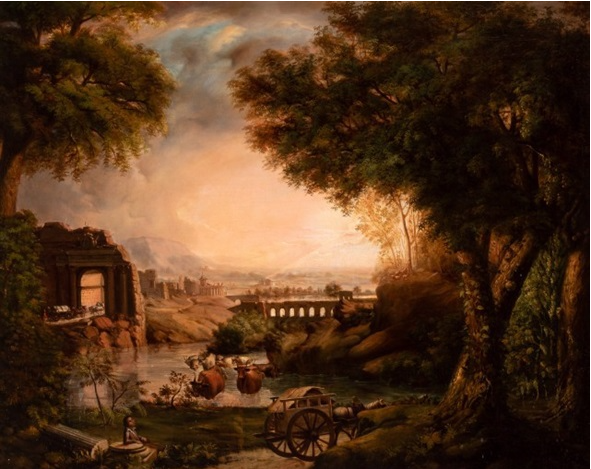The painting depicts a picturesque countryside scene bathed in the warm golden hues of sunset. In the forefront, an old-fashioned cart with two large, rear wheels and various objects like vases or urns scattered around it. The cart appears to be preparing for market, reinforcing the rural setting. Adjacent to the cart is a large, lush, green tree with intricately detailed leaves that reach up towards the sky. The scene is surrounded by numerous reddish-brown trees, creating a rich, autumnal palette. 

Off in the distance, you can observe the remains of ancient, Roman-like ruins hinting at a past civilization. There is also a small road beginning near the cart, along which a carriage, possibly horse-drawn, travels toward a nearby town. The road leads to a bridge and a series of walking paths. To the left of the scene, there's part of a building visible, perhaps a house with a window suggesting someone might still reside there. Beyond the town, a mountain range looms, further enhancing the depth of the scene. The sky above, painted with the soft glow of either a rising or setting sun, adds a final touch of tranquility and beauty to this detailed and serene countryside landscape.